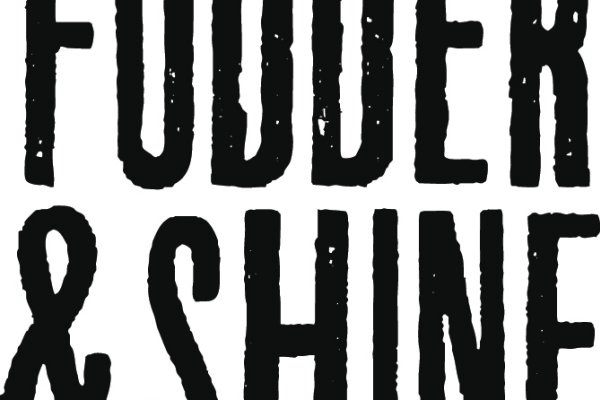The image depicts a graphic art logo featuring the words "FODDER" and "SHINE" in capital letters. Both the top portion of "FODDER" and the bottom portion of "SHINE" are partially cut off, giving the text a fragmented appearance. The font is black with a rough, rugged texture, and it is detailed with white blotches resembling driplets or sprigs of paint scattered across all the letters, except the "&" symbol and possibly the letter "E." The background of the image is white, suggesting that this design could be used for various graphic applications, including t-shirts.